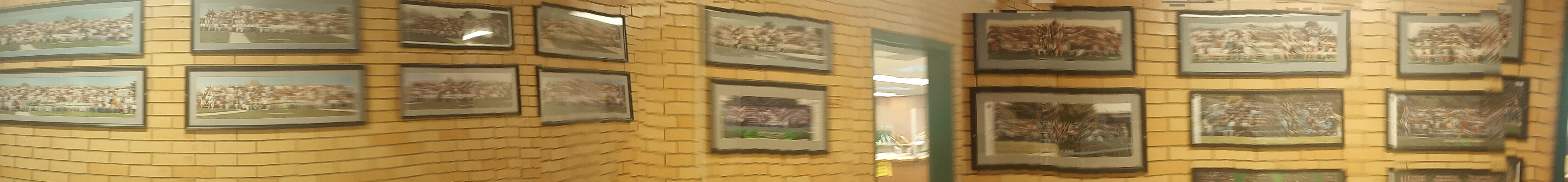The image depicts a long, panoramic view of a sandy-colored brick wall with a warm, yellowish tone. Mounted on this wall are numerous rectangular, horizontally-oriented framed photographs. The total count of frames includes eight on the leftmost wall, two in the center, and six full ones on the rightmost wall, though if partial frames are included the count is eight on the right. These frames contain blurry images that seem to depict group photos, possibly of school classes or sports teams, judging by the uniform arrangement and the reflection of fluorescent lights. Between the center and right portions of the wall, there is an archway with a green-painted interior, leading to what appears to be an office with a counter visible beyond it. Despite the blurred details, the setting resembles a school hallway, characterized by its long, uniform stretch and the repetitive pattern of the displayed photos.